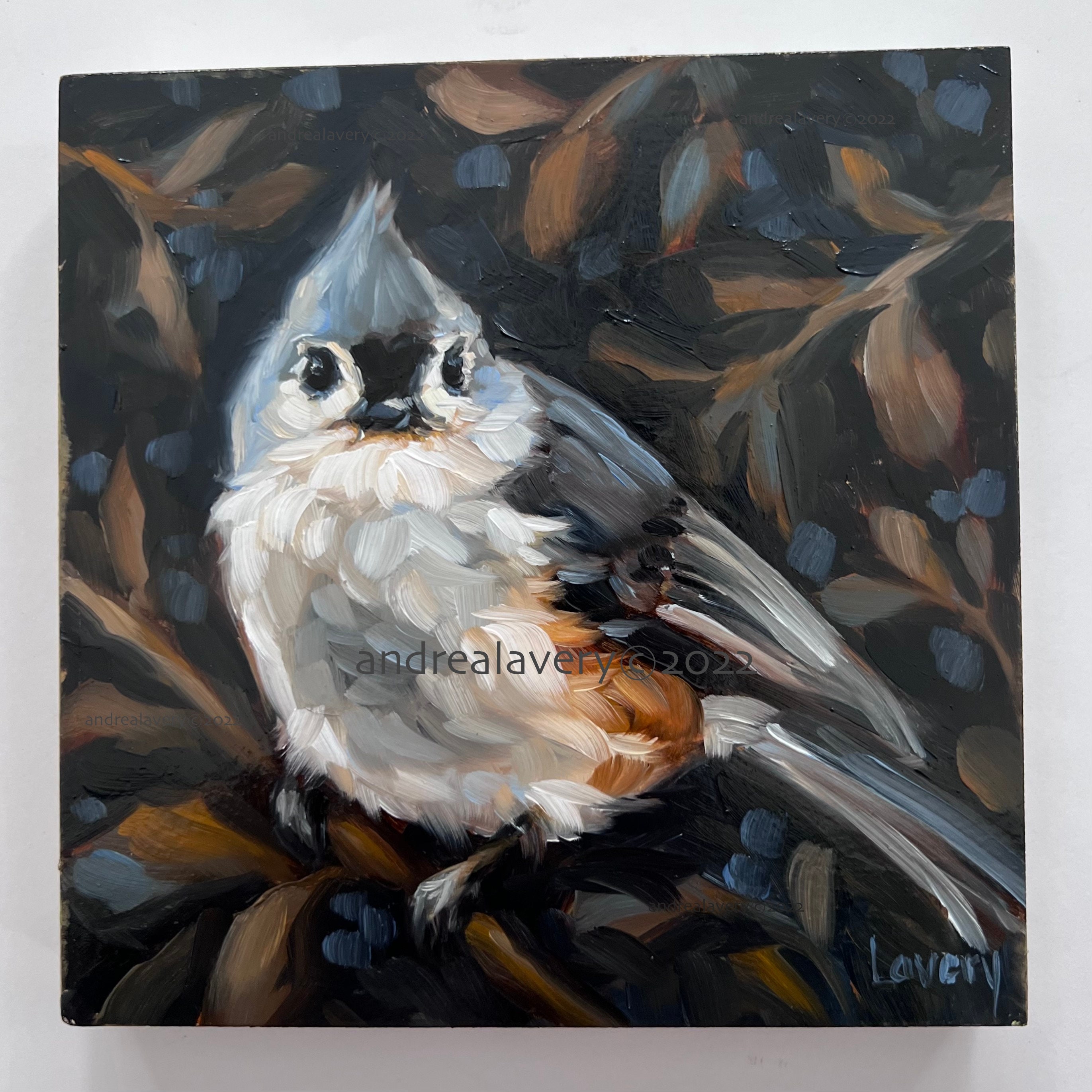This impressionistic painting features a small bird perched on a brown branch in the lower left portion of the composition. The bird's belly is white with rough brushstrokes that transition to a light gray, while the rear feathers are a light reddish-brown. Its wings and tail display various shades of blue, gray, and white; the tail has a blue top and gray bottom, and the wings blend blue and gray on the top right, tapering to white at the tips. The bird's head exhibits a rough crest, shaded in light blue to gray, with a small black beak and two black circles representing the eyes.

The background of the painting is comprised of black with brown twigs dotted with blue flowers, adding a delicate, naturalistic touch. This scene is framed by a grayish border, possibly indicating either a physical frame or the artwork's background setting.

In the bottom right corner of the painting, the artist's name, Lavery, is rendered in blue text. Additionally, across the bird's belly, rear, and wing, there is a small gray watermark that reads "Andrea Lavery © 2022." The meticulous brushstrokes and thoughtfully chosen color palette highlight the textured and dynamic nature of this watercolor or regular painting, showcasing the artist's skill and attention to detail.